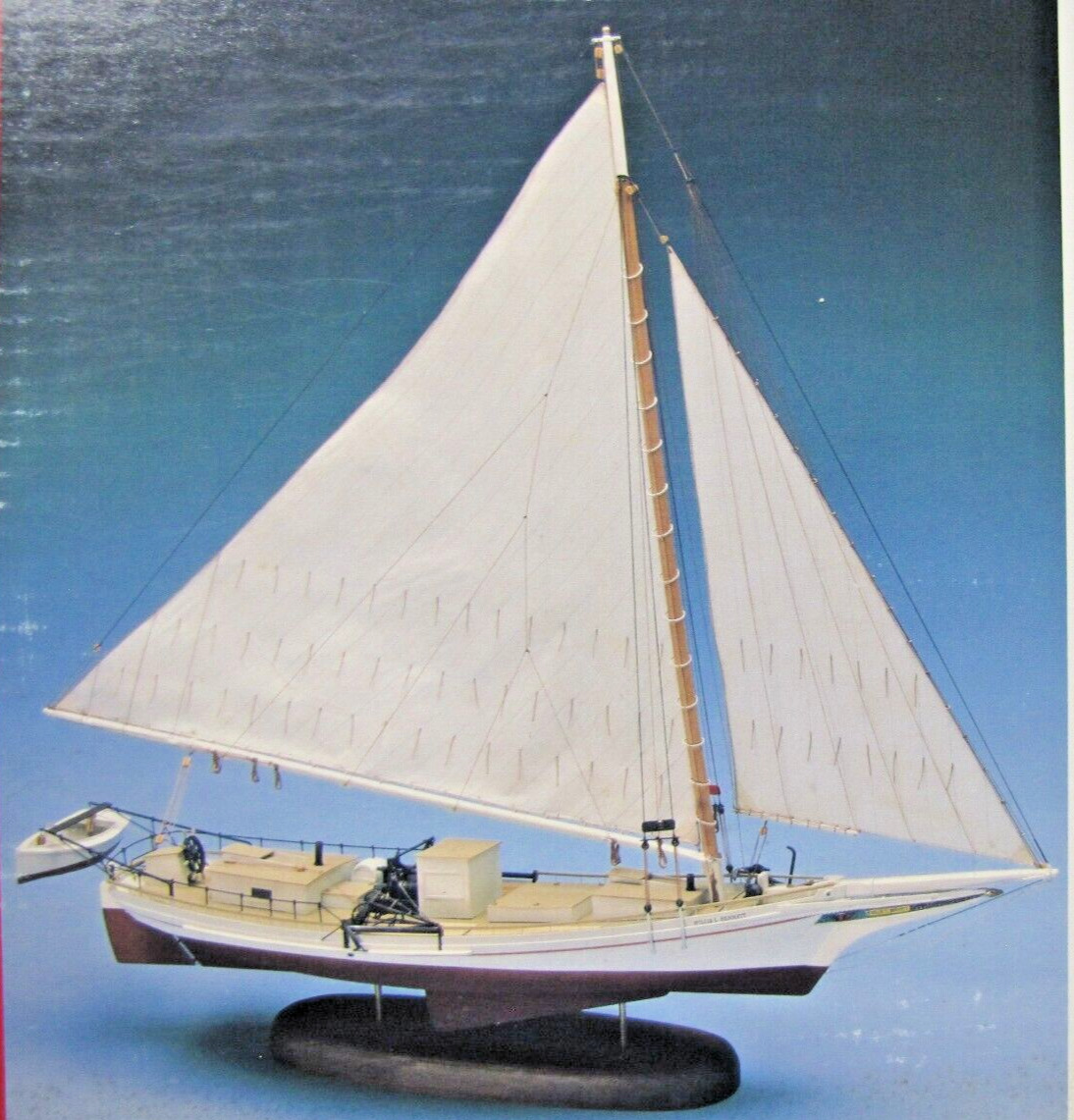This photograph showcases an intricately crafted model sailboat poised on a wooden base with dual metal supports, giving the impression of it gliding on water against a blue gradient background. The model features a distinct brown hull transitioning to a white upper section, complemented by a beige deck where a faint figure is visible. The sailboat is rigged with two prominent white sails: a large triangular main sail extending to the back and a smaller one at the front. Noteworthy details include a black railing around the deck, numerous lines for maneuvering the sails, and a dinghy securely attached to the stern. The presence of tan, black, and dark gray accents enrich the detailed model, highlighting different structures on the cabin and making it a vivid representation of a real sailboat.